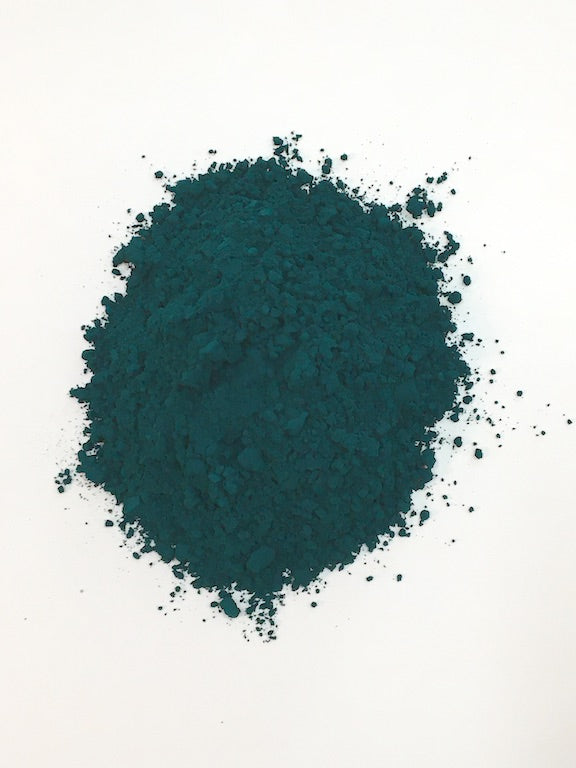The photograph depicts an overhead view of a mound of teal turquoise powder on an off-white background. The powder forms an oval-shaped pile, roughly two and a half inches by two inches in size. The mound is slightly chunky with clumps interspersed among finer grains. Stray grains of powder are scattered around the periphery of the main pile, especially on the right side. The dark blue-green hue of the powder suggests it could be used for something like cosmetics or possibly artistic materials, although its exact purpose remains uncertain. The image is vertically oriented, one and a half times as tall as it is wide, accentuating the contrast between the vibrant hue of the powder and the muted background.